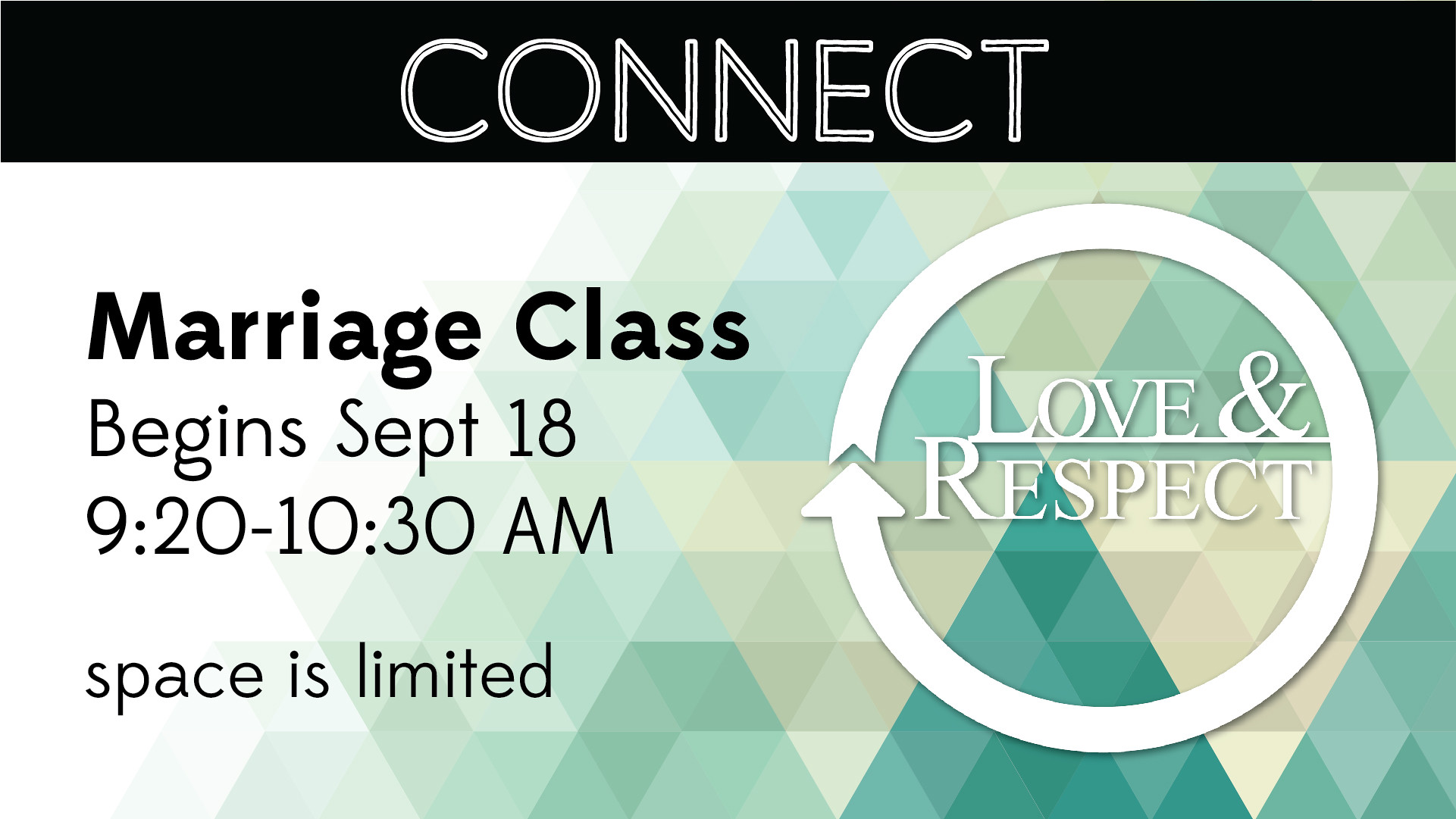This image is a detailed banner advertisement for an upcoming marriage class. At the top, there's a prominent black border featuring the word "CONNECT" in bold white capital letters. The main section of the banner showcases critical information about the class against a gradient background of geometric, green, and tan triangles, which transition from white on the left to a darker teal green on the right. The text, primarily in black, states: "MARRIAGE CLASS BEGINS SEPTEMBER 18th, 9:20 to 10:30 A.M. SPACE IS LIMITED." On the right side of the banner, a white circle with a subtle drop shadow contains the words "LOVE AND RESPECT," encircled by an arrow, symbolizing continuity and connection. The overall design employs a blend of black, white, light blue, brown, dark blue, and dark green colors, aligning the text centrally and artistically against the backdrop to create an engaging and informative visual announcement.